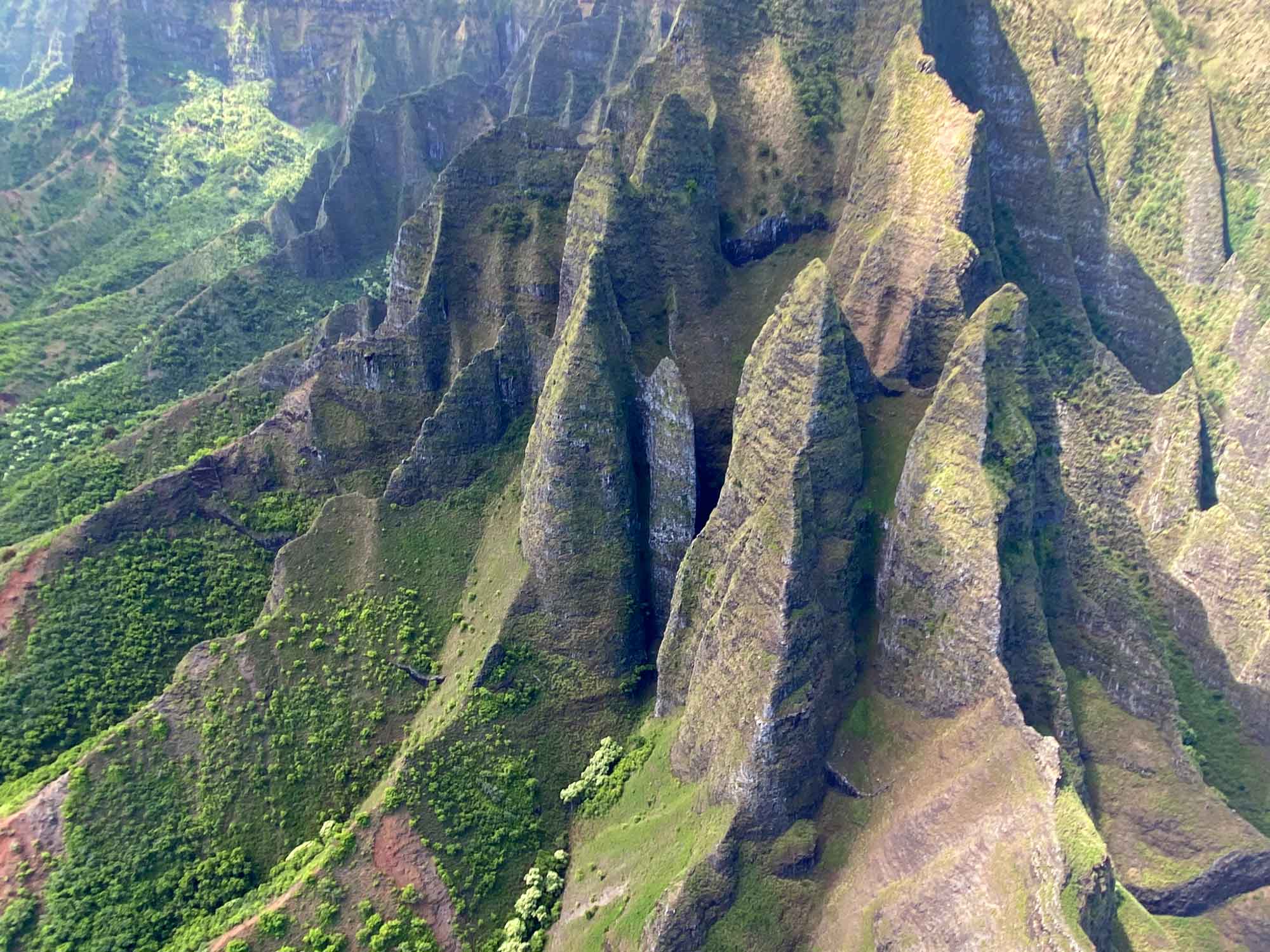The image is a detailed aerial photograph captured in landscape orientation. Dominating the right side of the frame are towering, pinnacle-style rock formations that rise steeply like cones with flat-edged faces, giving them a square appearance. These structures, primarily dark gray with a green, mossy film, culminate in sharp, pointy peaks. Among them, two near the center stand almost identical to each other. Behind these pinnacles, a sheer rock cliff climbs vertically, featuring patches of white and casting shadows on the adjacent rocks. The lower left of the image transitions to a gentler slope adorned with dense green vegetation, including round bushes and trees. The bottom portion of this slope is covered in vibrant greenery, while the upper left corner is highlighted by a bright spot of light illuminating the mossy terrain. The photograph encapsulates a blend of rugged, rocky peaks and lush, verdant growth, captured with the clarity and realism typical of drone photography.